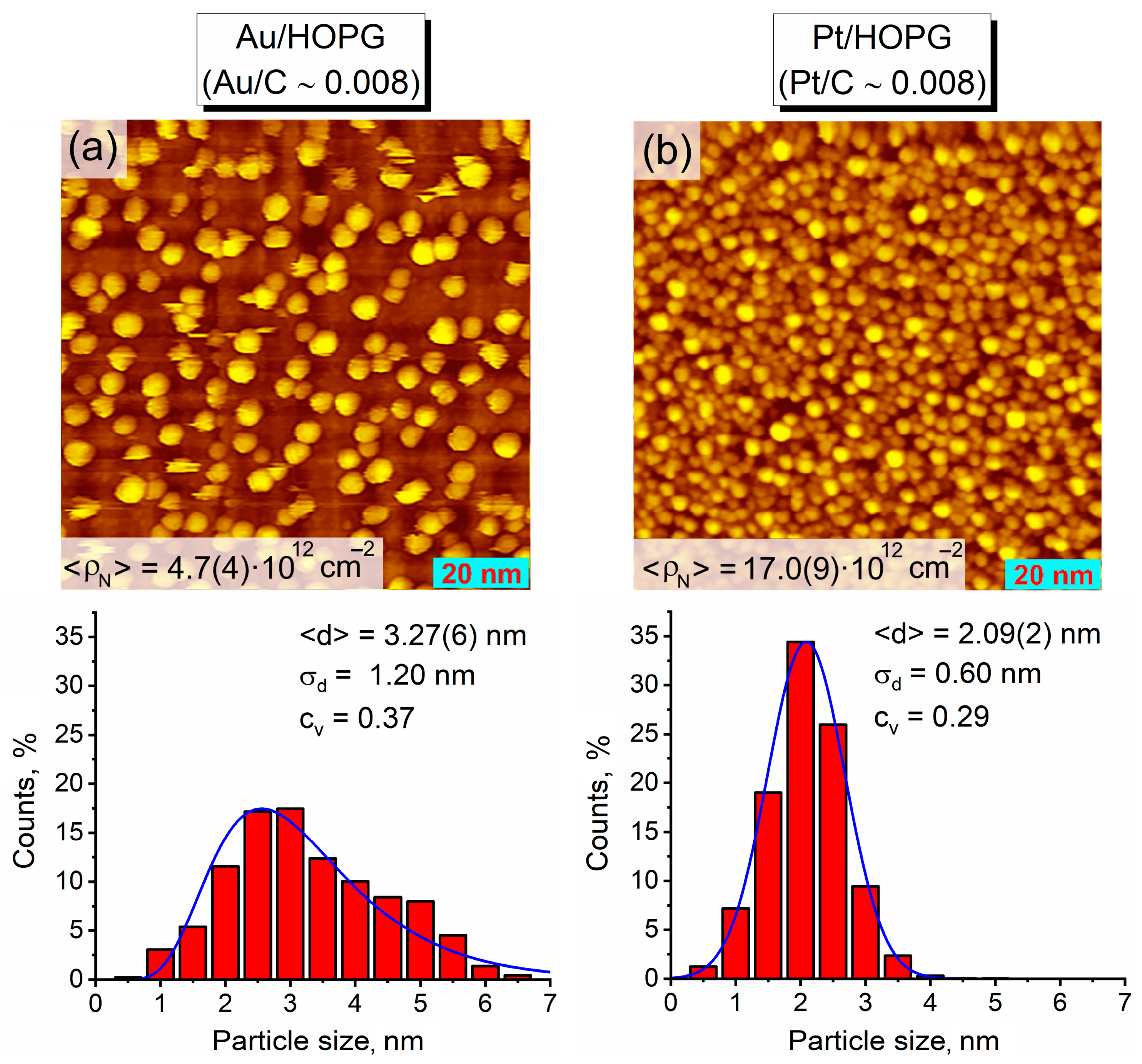The image displays two scientific charts labeled A on the left and B on the right. Both charts feature a brownish background densely covered with yellow dots resembling small spheres or pieces of corn. Chart A is titled "AU/HOPG, AU/C-0.008," while chart B is labeled "PT/HOPG, PT/C-0.008." The top sections of both charts are characterized by heavy yellow-orange and orange-red colors, with chart B showing a noticeably higher concentration of yellow dots compared to chart A.

Below each image, there are corresponding bar graphs. The vertical axis of these graphs represents count percentage, scaling up to 35%, and the horizontal axis shows particle size. In chart A, the particle sizes are less than 20%, resulting in a flatter and more gradual curve. Conversely, chart B shows a steeper curve with the bars rising higher, almost reaching the 35% mark, indicating larger particle sizes and a more concentrated distribution. The detailed labeling and differences in density and graph shapes emphasize the contrasts between the two sets of data.